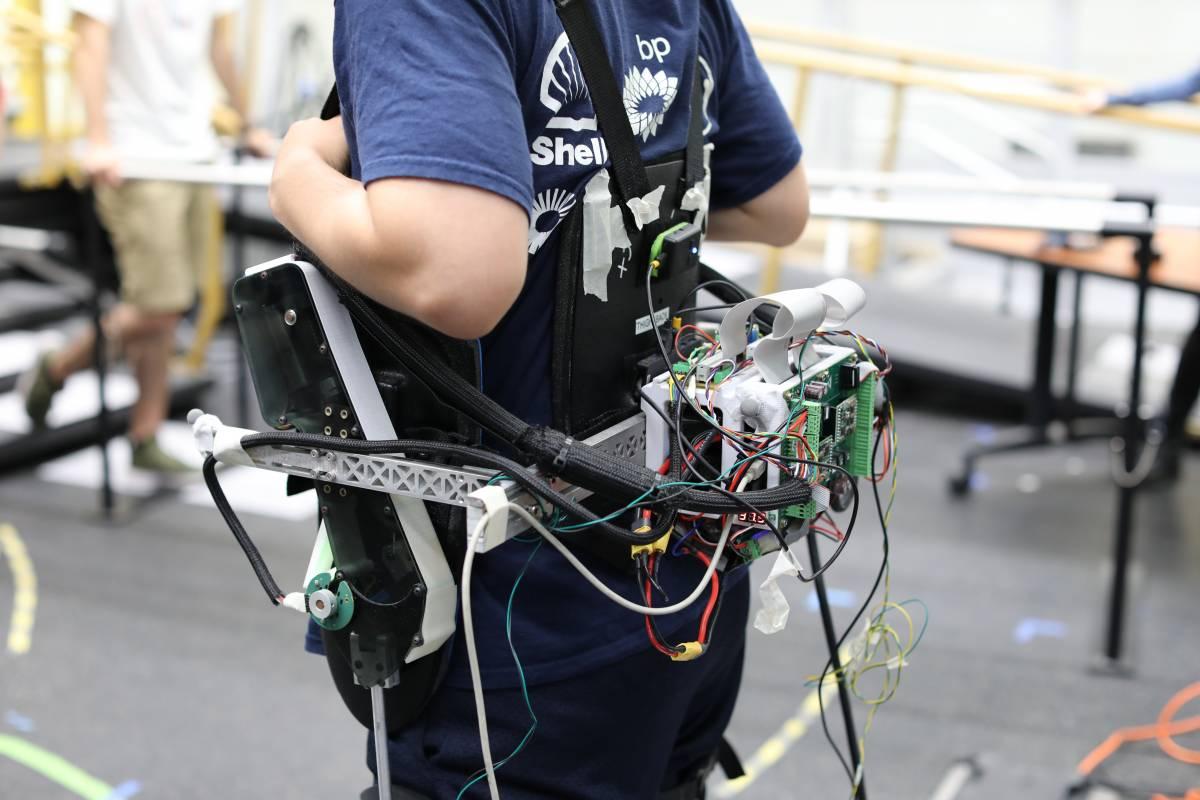In this realistic and detailed photograph, we see the backside of an individual wearing a sophisticated, experimental assisted walking device. The person, clad in a blue t-shirt with visible Shell and BP logos, and blue jeans, is facing away from the camera. The image zooms in to show only their torso down to the upper thighs. They are strapped into a complex apparatus with a large, green and white battery pack on their back, featuring an array of multi-colored wires—red, white, and black—dangling in various directions, indicating the device might still be in a prototype stage. This mechanical contraption includes a harness around their shoulders and multiple components monitoring different functions, attaching around their waist and legs. Surroundings are blurred, but distinguishable; to the left, an individual in a white shirt and tan cargo shorts, and on the right, partial glimpses of another person's arm and leg. Orange cables and a rolling table are also subtly visible in the backdrop.